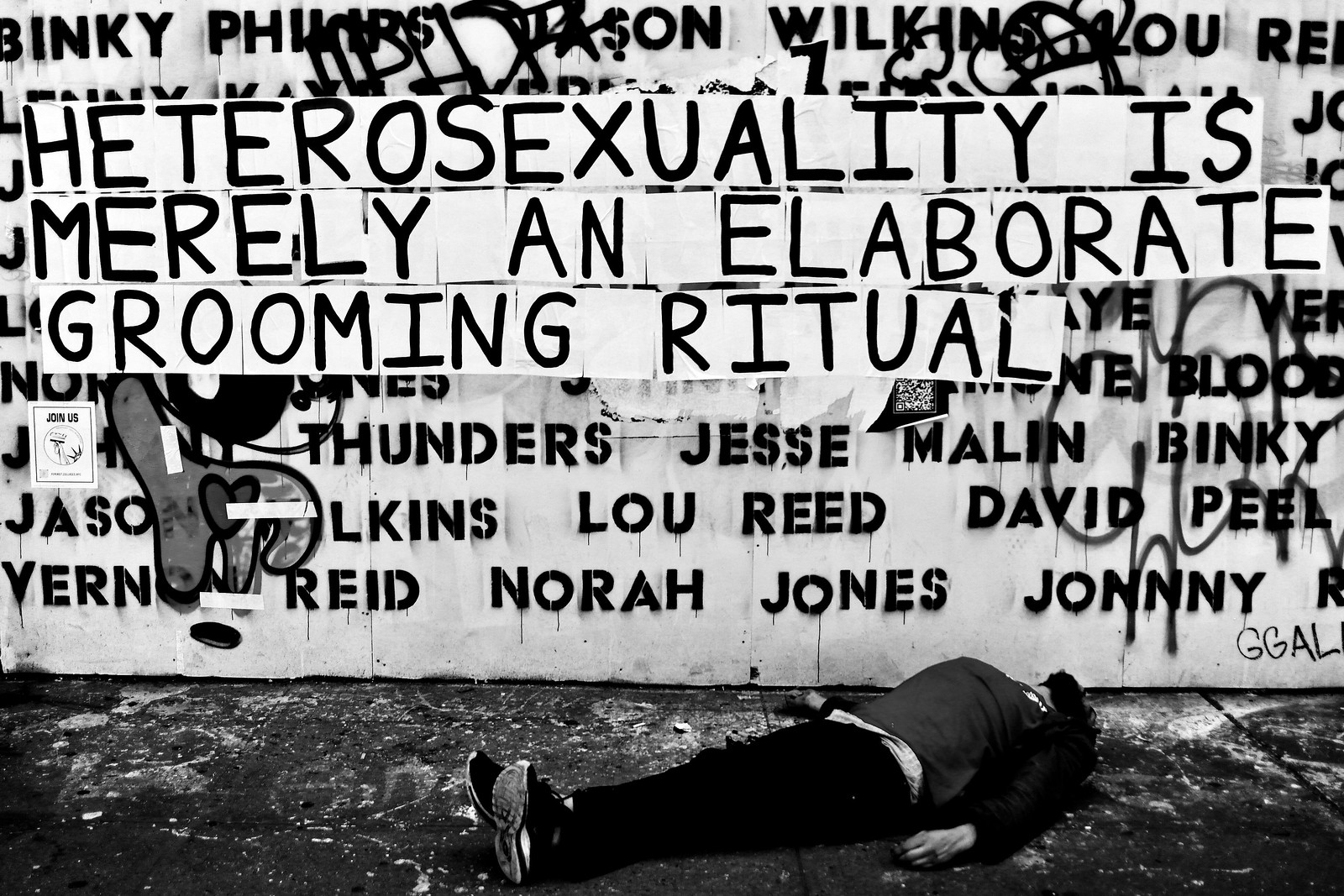The black-and-white photo captures a wall adorned with graffiti, prominently featuring the phrase "Heterosexuality is merely an elaborate grooming ritual" in black letters. Below this striking message, the wall is covered with various names, including those of renowned artists Lou Reed and Nora Jones. Lying on the concrete ground which is stained with spilled paint from the graffiti, there is an indistinguishable figure. The person, clad in dark pants, a dark shirt, and black tennis shoes, appears motionless, leaving their state of consciousness ambiguous – they could either be alive or deceased. The scene suggests a possible protest conveyed through the graffiti, adding a layer of social commentary to the image.